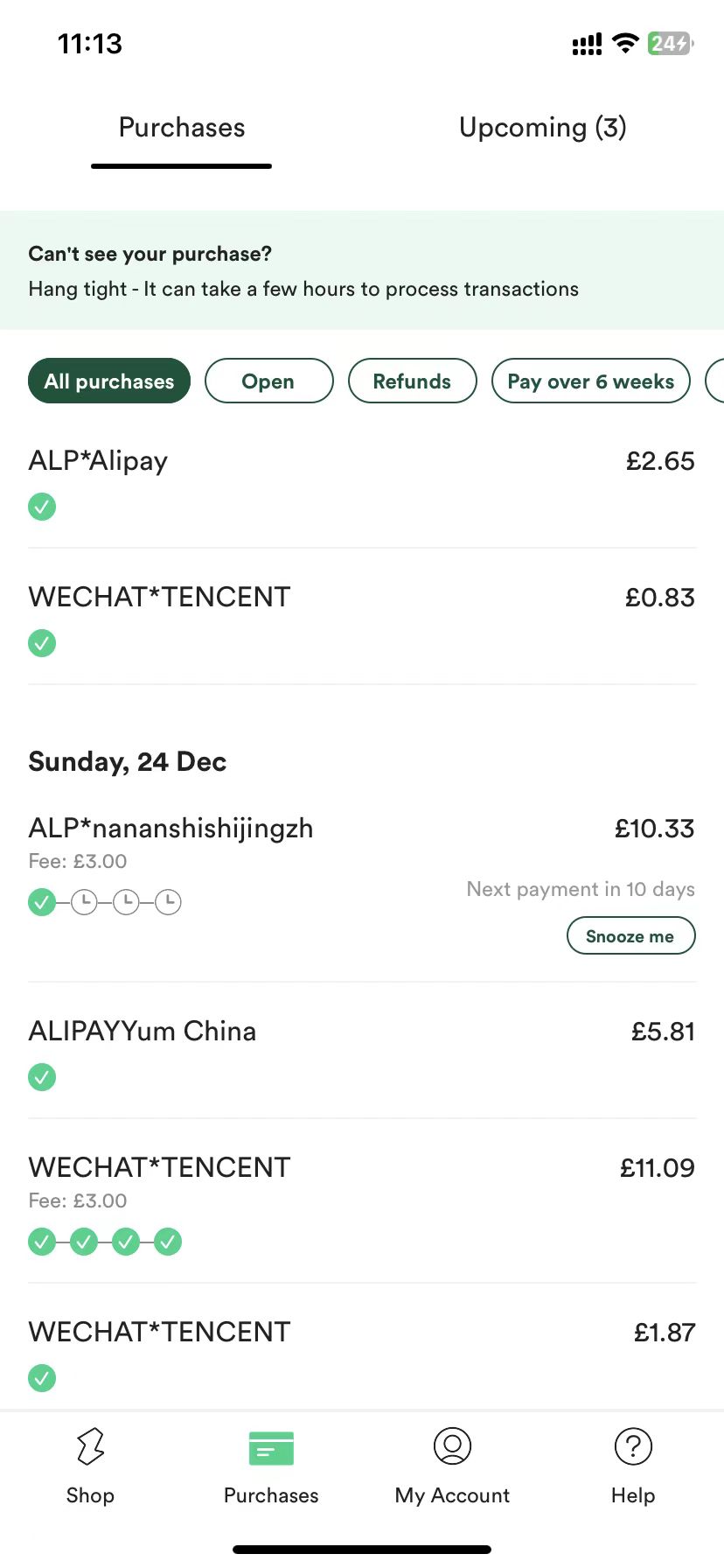This image is a screenshot taken from a mobile phone displaying what appears to be a payment system interface, likely from an app such as Alipay or a similar service.

The interface has a predominantly white background. At the top left corner of the screen, the number "1113" is displayed, alongside signal bars for both phone and Wi-Fi connectivity, which indicate "24+".

Below this, on the left side of the screen, there are sections labeled "Purchasing" and "Upcoming (3)". A blue rectangular bar at the top contains the text: "Can't see your purchases? Hang tight. It can take a few hours to process transactions."

Underneath this notification, there are several buttons, each with a different function:
- The "All Purchases" button, which is green.
- The "Open" button, which is white.
- The "Refunds" button, which is white.
- The "Pay over six weeks" button, which is white.

Following these buttons, a series of transaction entries with check marks are listed:
- Entry for Alipay with a checkmark indicating £2.65.
- Entry for WeChat (Tencent) also with a checkmark showing 83 pence.
- An entry dated Sunday, 24 December, detailing an Alipay transaction labeled "Nana Manshiptangzili" with a fee of $3 and a total of £10.33. It also notes that the next payment is due in 10 days.
- Another Alipay transaction for Yum China amounting to £5.81.
- A WeChat (Tencent) transaction with a fee of $3 amounting to £11.09.

Further down, there are four more transactions each indicated by a check mark:
- Another WeChat (Tencent) transaction for £1.87.

At the very bottom of the screen, several icons are displayed for navigating different sections:
- A green "Shop" icon.
- A "Purchases" icon.
- A "My Account" icon.
- A "Help" icon.

This detailed description provides an extensive breakdown of the elements and transactions displayed in the screenshot.